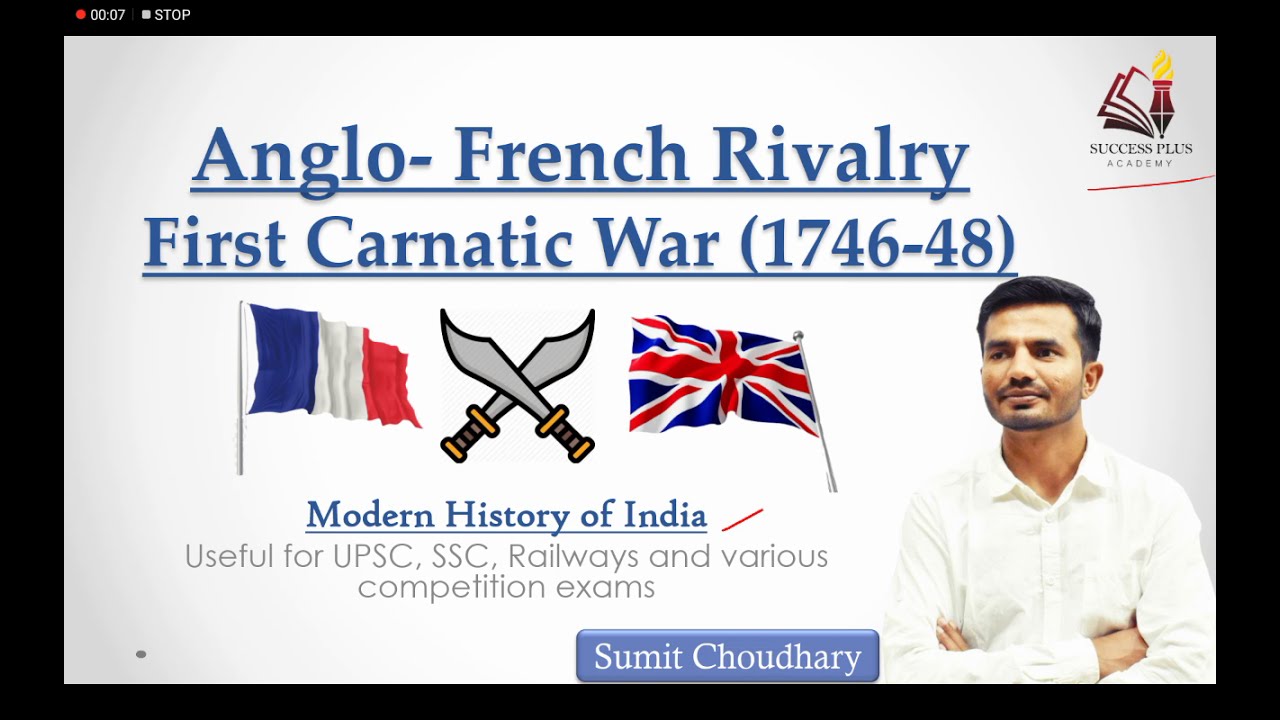The image is a screenshot of a website, primarily white in color with blue lettering. At the top right-hand corner, there is a logo featuring a red book and a lantern, labeled "Success Plus Academy." Prominently across the middle in blue letters, it reads "Anglo-French Rivalry, First Carnatic War (1746-48)." Below this headline are two flags: to the left is a blue, white, and red horizontal striped flag (French flag), and to the right is the British flag (Union Jack). Between the flags, two crossed swords enhance the visual. Further down, it states "Modern History of India," and notes that the content is useful for UPSC, SSC, Railways, and various competition exams. Below this is the name "SUMIT CHOUDHARY" next to a picture of a man with short dark hair, a dark beard, and mustache, dressed in a white button-down shirt, standing with his arms crossed and looking slightly to his right. The overall style merges an informational graphic with photography within a video-still-like frame, complete with a counter, red light, and the word "stop" in the top left corner.